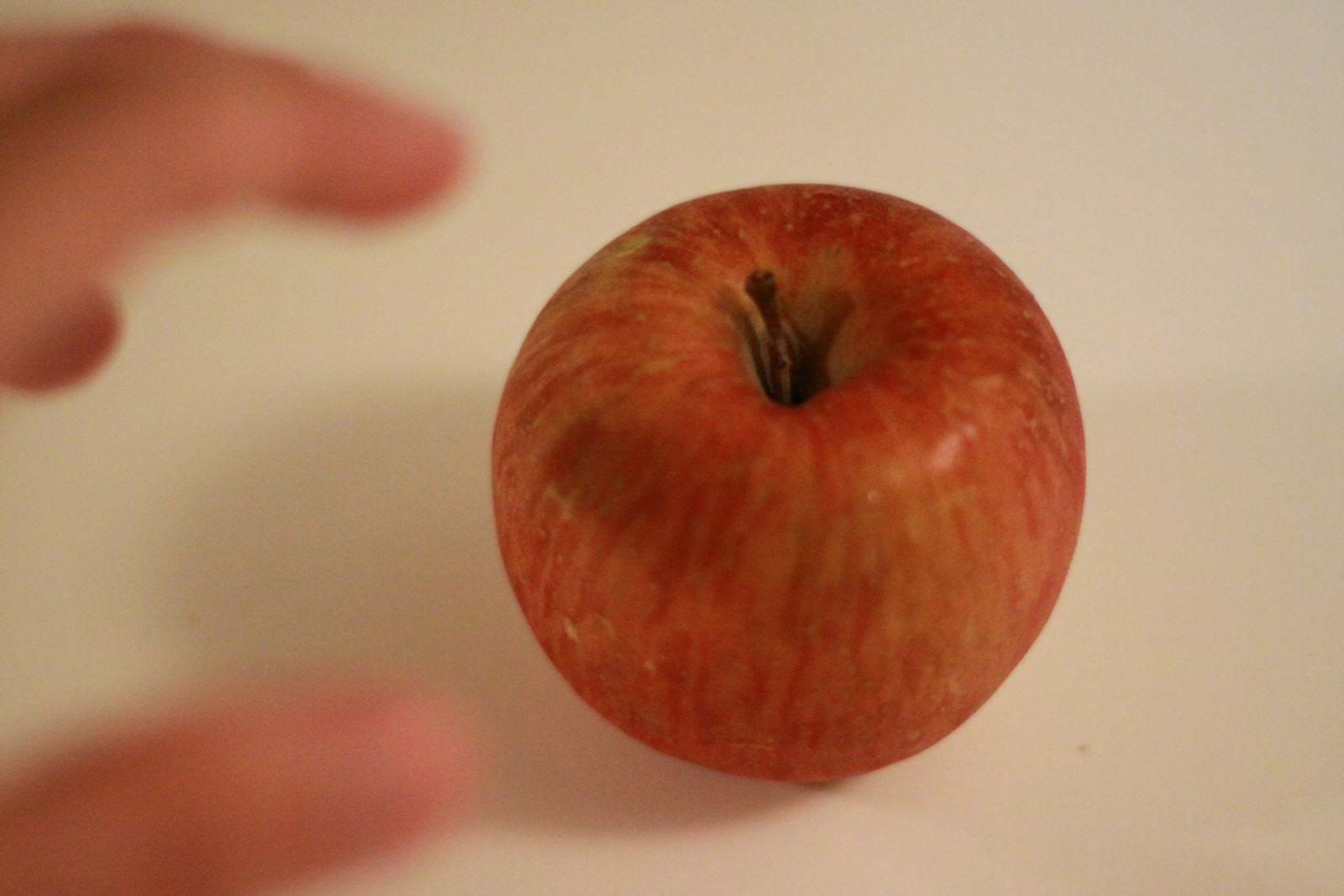A close-up photograph of a red apple, which is not fully crimson but exhibits varied shades of red. The apple has a couple of stems protruding from it. In the background, there is a hand reaching towards the apple, though the hand is blurred and only the fingertips of the fair-skinned person are visible. The apple casts a distinct shadow below it on the surface it's resting on, adding depth to the image. The stems of the apple also create subtle shadows on its glossy skin, enhancing the texture and detail of the fruit.